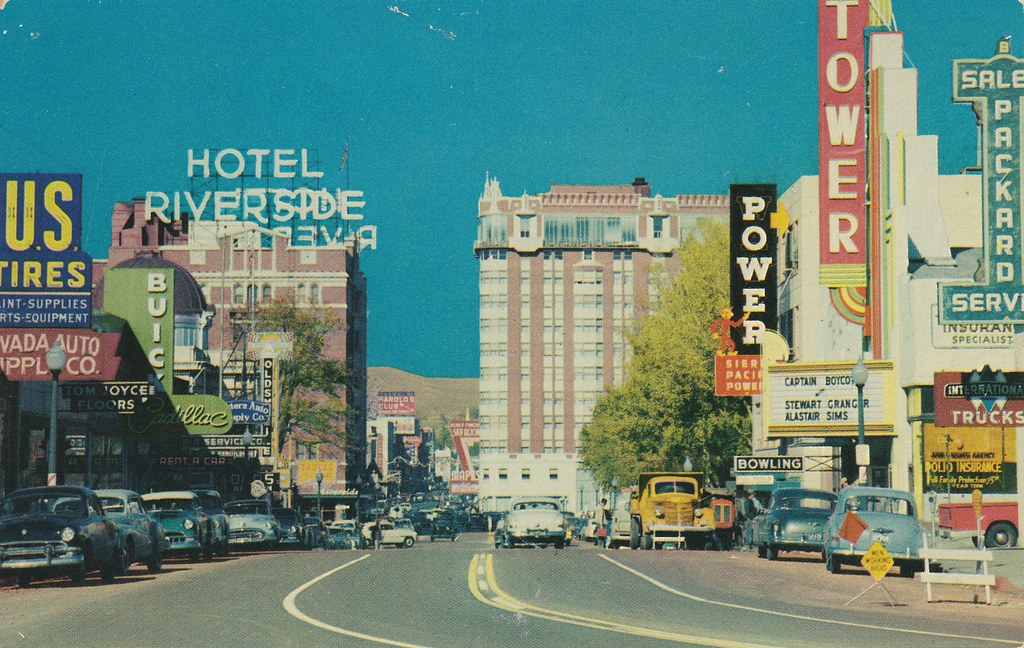This photograph appears to be taken in a cityscape dating back to the 1960s or 1970s, characterized by its antiquated grading and wear, as indicated by small white markings that show the image's age. Dominating the left side of the street is Hotel Riverside, a prominent building with a distinctive sign. The street is filled with a variety of older model cars, including several that resemble Volkswagen Beetles, both on the road and parked along the curbside. On the right side of the image, notable signboards with retro fonts advertise various businesses, including a movie theater named Tower, displaying a marquee that partially reads "Captain Boycott" and mentions actors Stuart Kringer and Alastair Sims, though some parts are obscured by a streetlight. Other signs on the right include those for a bowling alley, international trucks, and a business offering Packard Services. The road itself is grey with a painted yellow line in the center and white side markings, contrasting with the clear sky above. Another sizable building similar to Hotel Riverside stands near the middle-right of the image, adding to the city's layered, bustling ambiance.